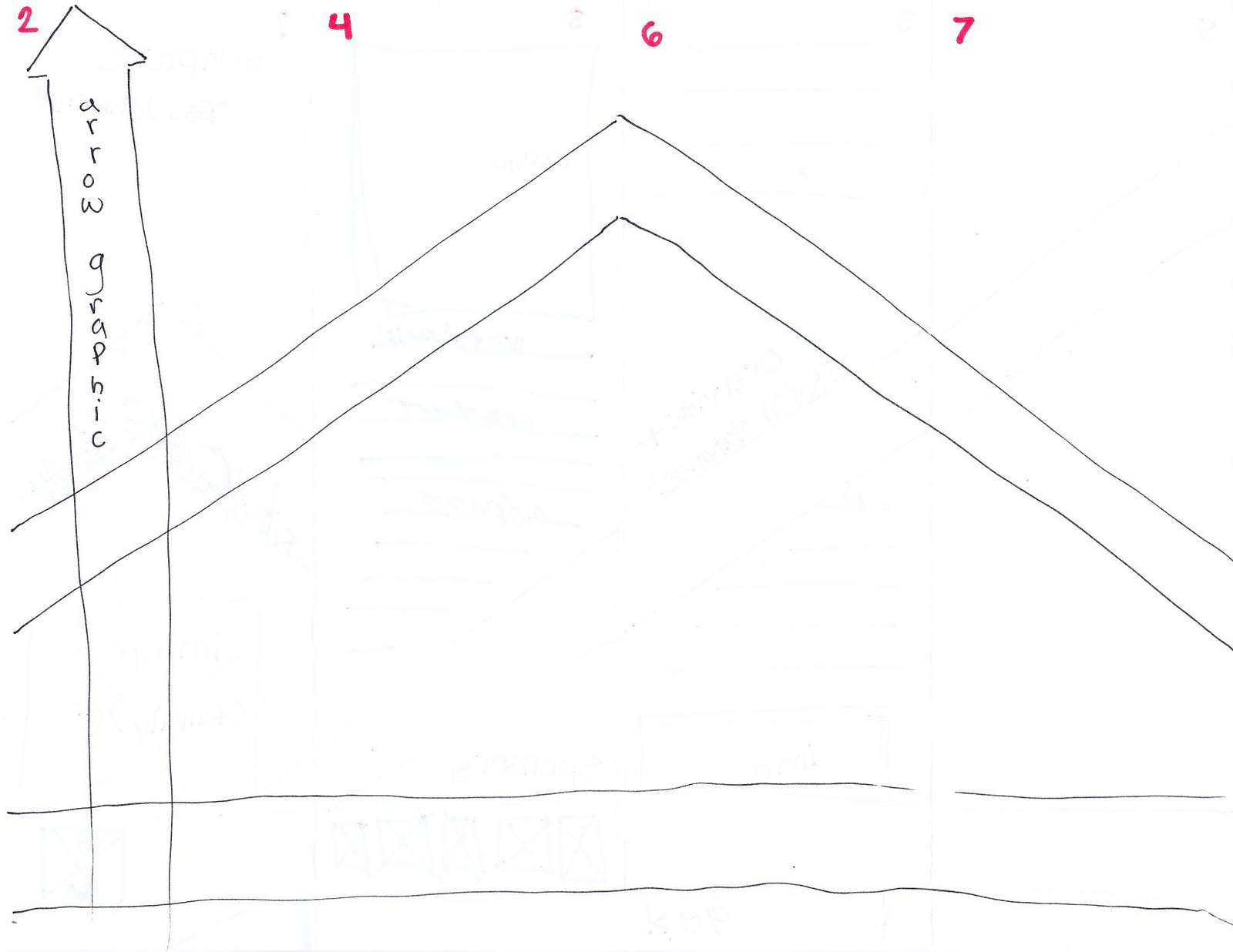The image displays a complex diagram featuring a series of elements. At the top of the image, red numbers—2, 4, 6, and 7—are arranged from left to right. The number '2' is located in the top left corner, while '7' is slightly off-center towards the right. Below these numbers, the diagram features a set of bold black lines, including a prominent vertical arrow extending from the bottom to the top of the image. This arrow, labeled "aero graphic" in vertical text, culminates in a pointed arrowhead.

Intersecting this vertical arrow is a large, triangular shape formed by lines extending from the sides of the image towards its center. Another similar triangular formation is mirrored below this intersection. Additionally, near the bottom of the diagram, two horizontal lines cross the image, intersecting with the vertical arrow on the left-hand side.